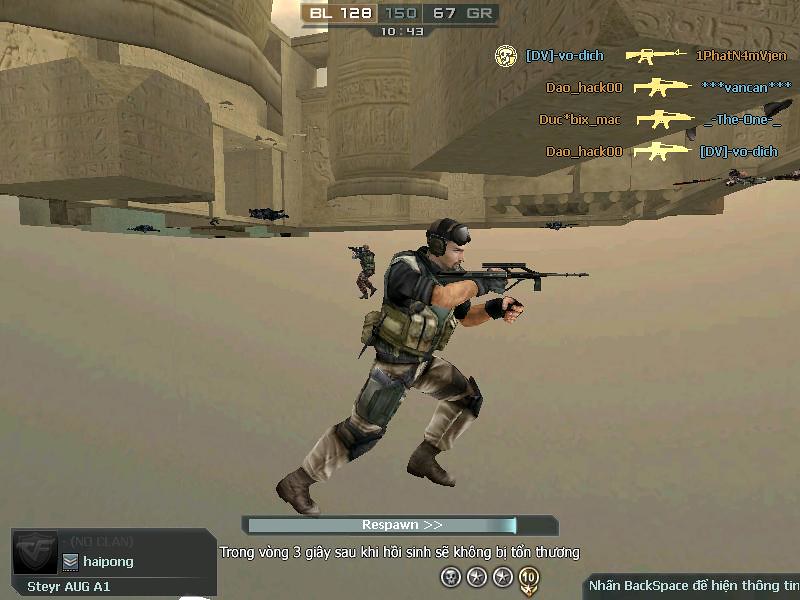In this screenshot from a video game, a soldier stands dead center, dressed in an army outfit consisting of black and brown fatigues, a black helmet, a utility belt along the waist, and black knee pads over khaki pants. The soldier is pointing a gun from right to left, looking off into the distance to the right. The surrounding environment is predominantly tan and brown, with sandy ground and tan buildings that evoke a desert or war-torn setting. 

In the background, a stone building with ancient carvings adds to the atmosphere. Another soldier can be seen in the distance, further emphasizing the game's warzone theme. Various game HUD elements are visible: in the top left, there are yellow weapons icons with red or blue writing. Numerical data in white font over different colored borders (e.g., "BL 128 150 67 GR 10 43") appears scattered across the screen. In the lower part of the image, a rectangular "respawn" timer is displayed, alongside non-English text "n-h-a-n d-e-h-i-e-n t-h-o-n-g-t-i-r," a skull, a star, and the number 10 in gold. The lower right corner shows additional unreadable white text in an unknown language, further contributing to the chaotic and immersive battlefield atmosphere.